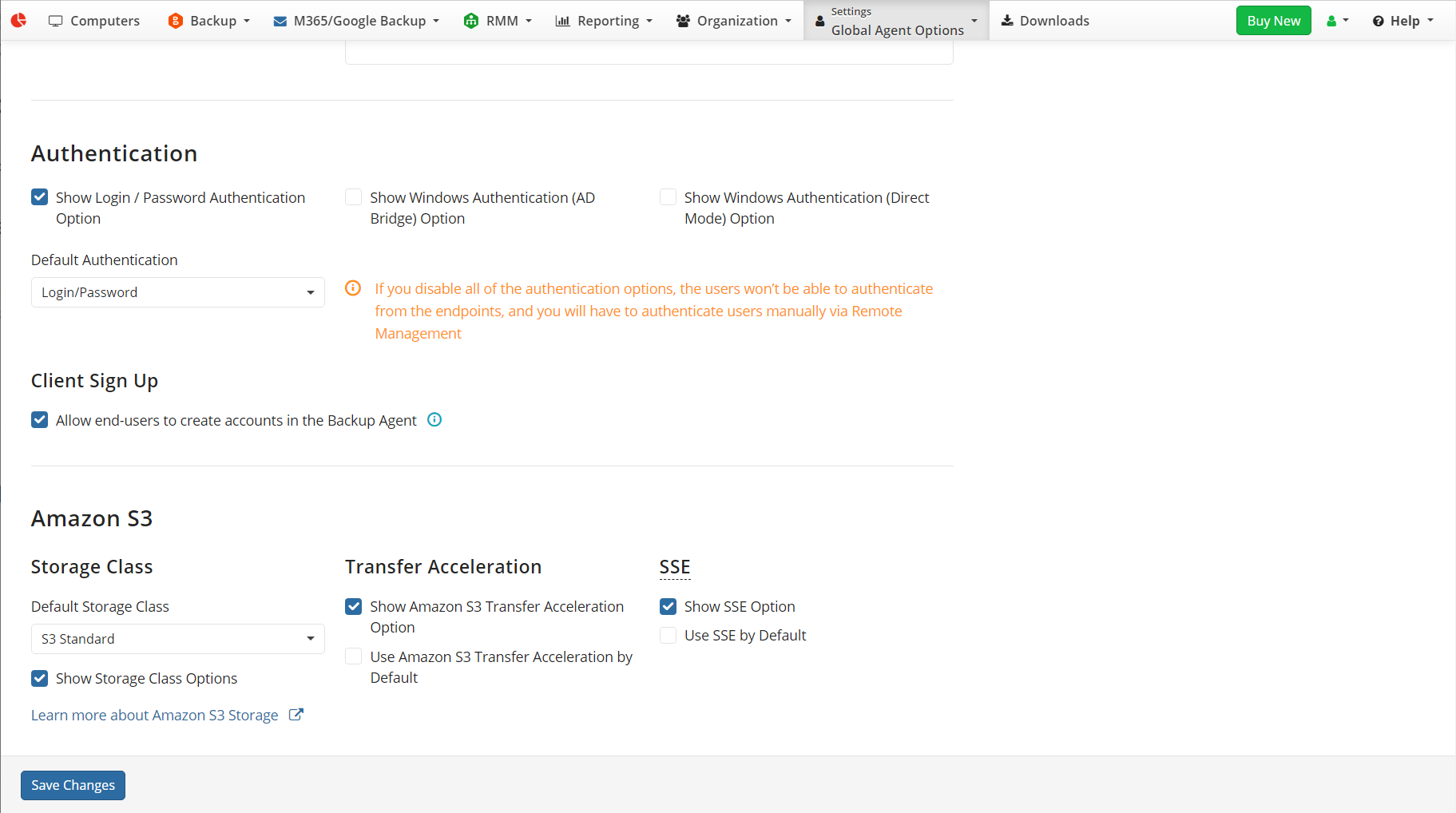The image depicts a computer screen interface related to backup management using services like Microsoft 365 and Google Backup. The user is navigating through Remote Monitoring and Management (RMM) options with various authentication and organizational settings.

The interface features several important elements against a predominantly green background with the phrase "Buy New." A user question is highlighted with "?" and "Help." The interface is largely white with notable blue boxes containing options and settings.

One section shows a blue box with a white checkmark labeled "Show Login/Password Application" and "Default Authentication Login/Password." Another highlighted option is "Show Windows Authentication," presented twice. An orange alert box warns, "If you disable all the authentication options, users won't be able to authenticate from the endpoints. You must authenticate users manually via remote management."

Additional settings include options for "Client Sign Up" where end users can create accounts in the backup agent. Another blue box mentions "Amazon S3 Storage Class," with the default set to "S3 Standard." There are options to "Show Storage Class Option" and learn more about "Amazon S3 Storage," including information on "Transfer Acceleration." The interface indicates an option to "Use Amazon S3 Transfer by Default" and shows a setting for "SSE" (server-side encryption).

Finally, user actions include "Save Changes" and "OK," both noted by a panelist, while the background features a simple instruction "Swipe." 

Overall, the screen is filled with a comprehensive array of customizable options and settings enhancing the management of backup processes and user authentication protocols.